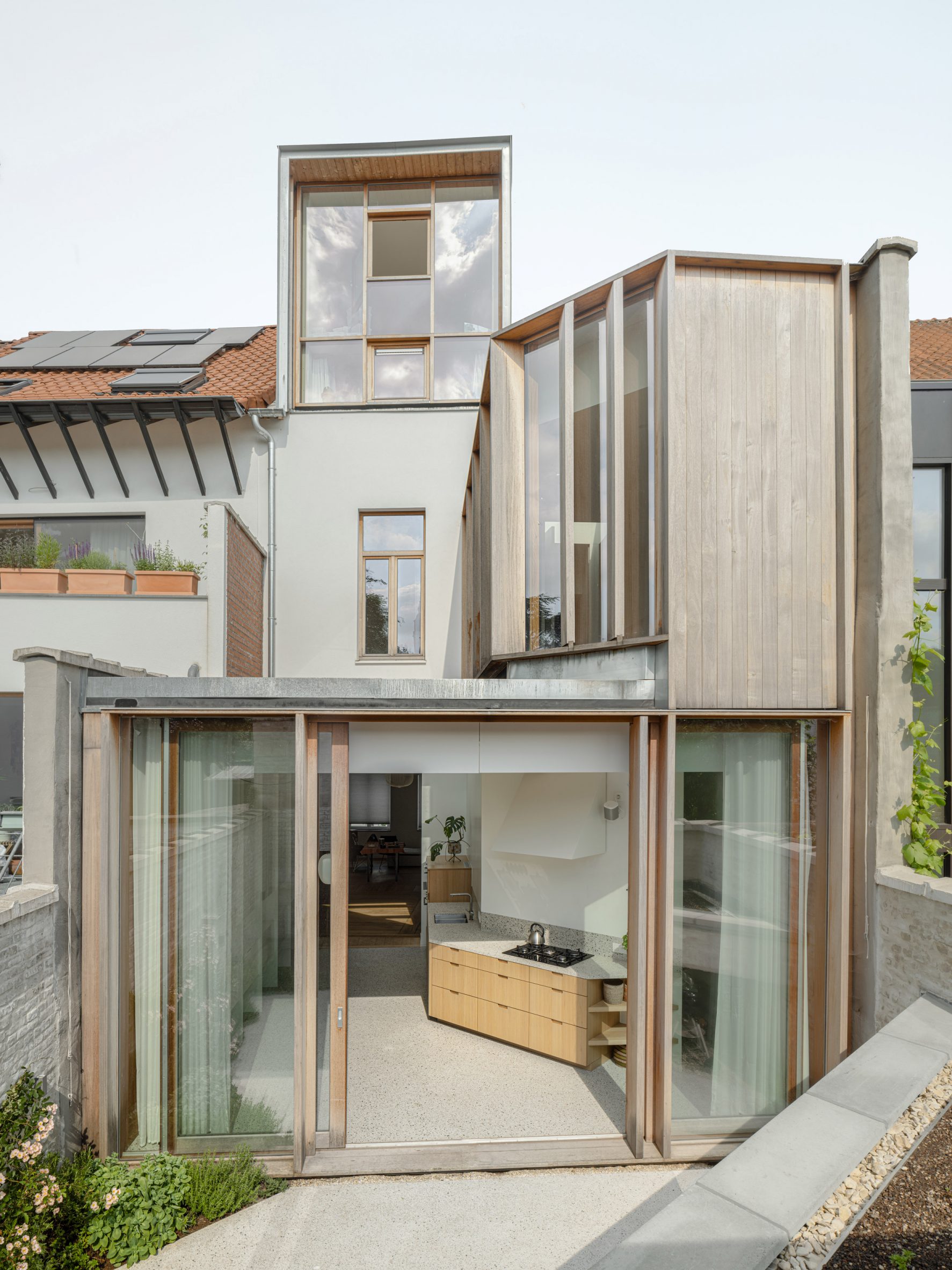This digital image depicts a strikingly flawless, modern house. The building itself is predominantly white with distinctive wooden sections on the upper right corner, complementing its orangish-colored roof adorned with solar panels. The house features an abundance of large, elongated windows on the left side, and a series of glass windows and sliding doors on the lower level which give it a very square and modern appearance.

Inside, you can see brown cabinetry and what appears to be a sink area. The interior, visible through the expansive windows, reveals a wooden drawer system and a black section with a curved item, hinting at a possible sink. Further inspection shows more rooms and windows on the higher levels, indicating a multi-story structure.

At the very bottom of the image, a small detail of landscaping is noticeable. On the left, there are some shrubberies while the middle section at the bottom reveals a sidewalk. The bottom right showcases another level with stones, pebbles, and dirt, suggesting that the picture might be captured from an elevated perspective.